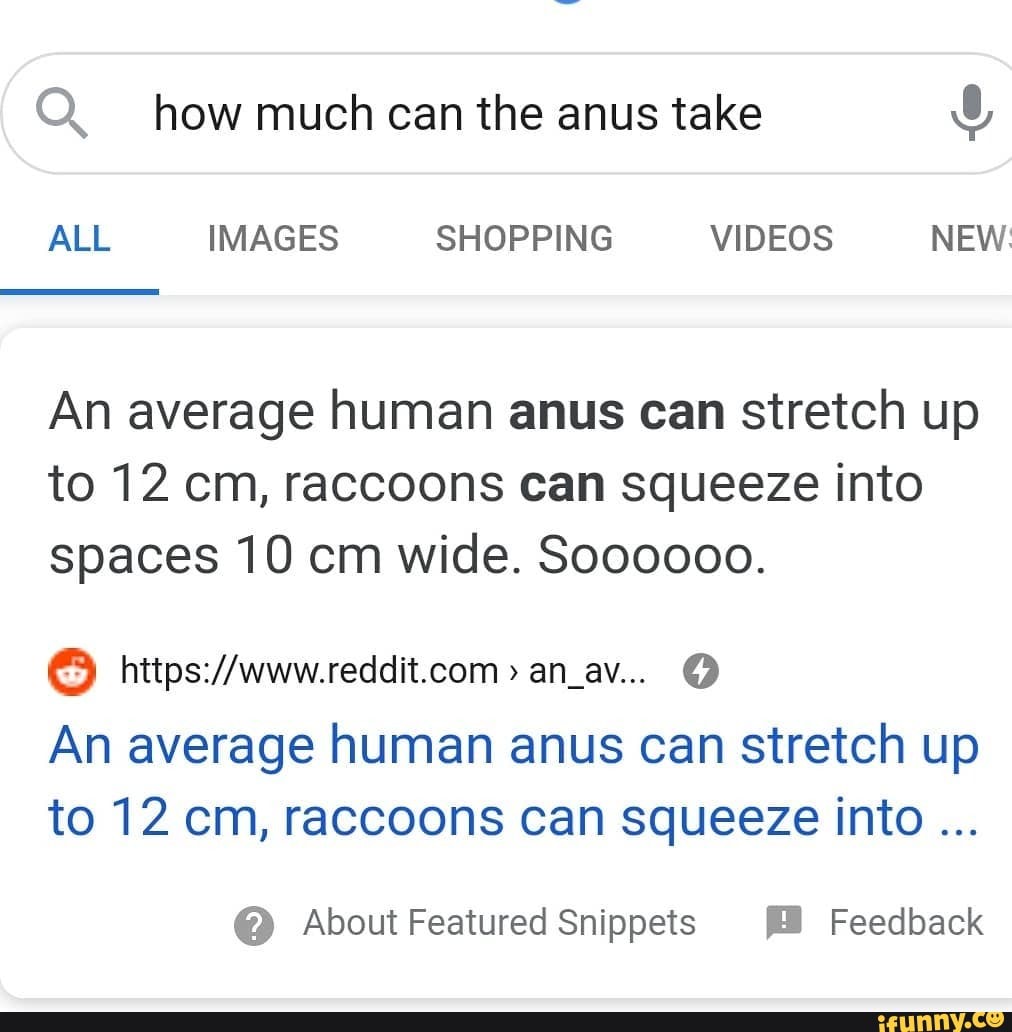The image is a screen capture of a search engine results page with a white background. Dominating the top portion of the image is a large, elongated search box featuring a gray search icon on the left and a microphone icon on the right. Inside the search box, the query is visible: "how much can the anus take."

Directly beneath the search box are the display options for the search results. The word "All" is highlighted in blue, followed by other options such as "Images," "Shopping," "Videos," and "News."

The search results are displayed in dark gray text below these options. The top result reads: "An average human anus can stretch up to 12 centimeters. Raccoons can squeeze into spaces 10 centimeters wide."

In the lower right corner of the image, there is a blue rectangular bar with yellow text indicating a watermark or branding from the website "ifunny.co."